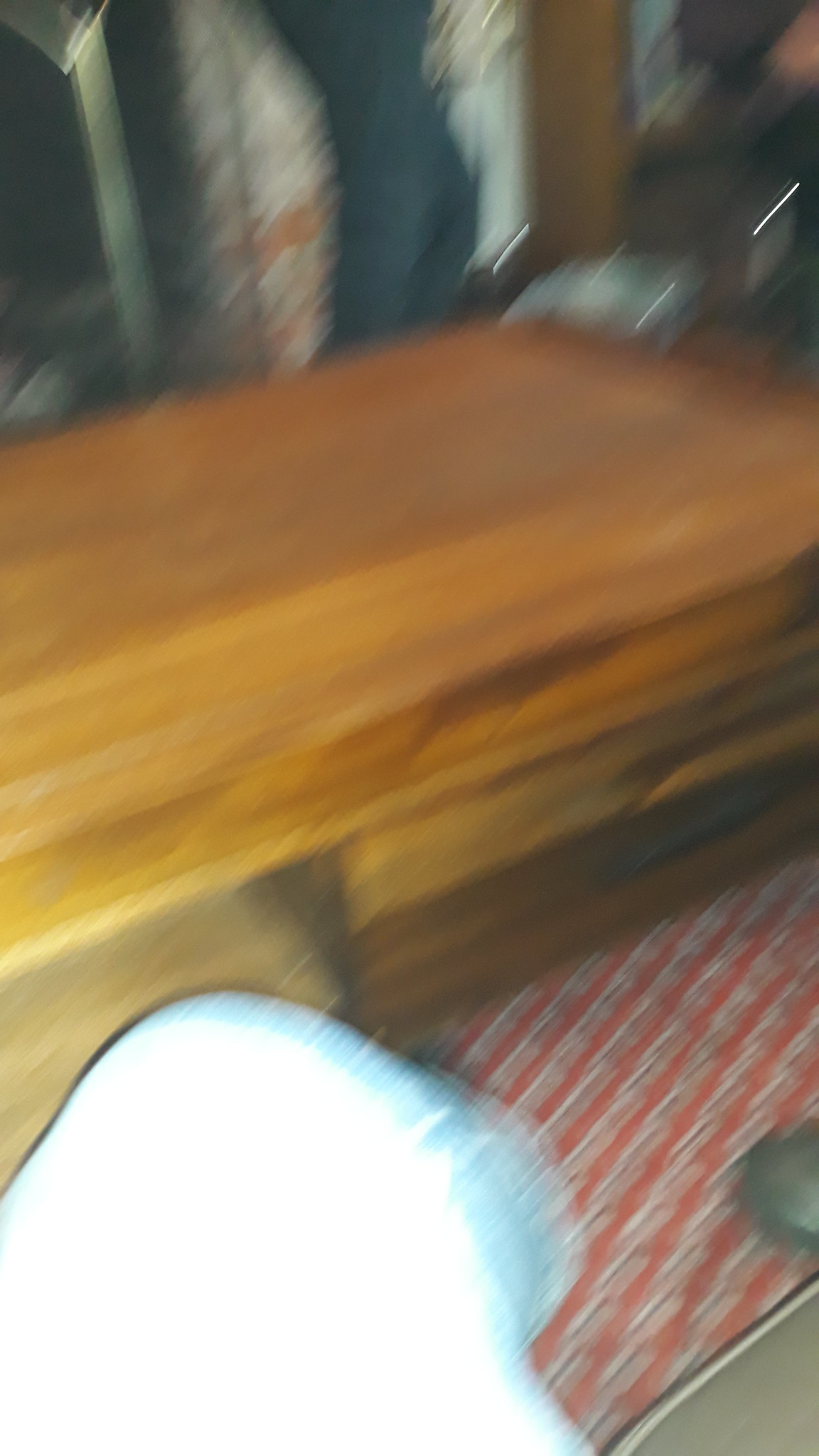This image appears to be a very blurry photo taken inside someone's house, showing a leg clad in light blue jeans positioned as if the person is sitting down. The leg is in the lower section of the frame, and the foot rests on what seems to be a patterned rug in shades of white, red, and black. There's a large light-brown wooden piece of furniture, likely a coffee table or a desk, in the foreground. In the bottom right corner, another person's foot with a black shoe is partially visible. The background features a cluttered scene that includes a wooden dresser with possibly one drawer at the bottom. Clothes hang above the dresser, including items that are long-sleeved and appear to be coats or thick garments; one garment is white with some orange, another is blue, and there are black and whitish items as well.